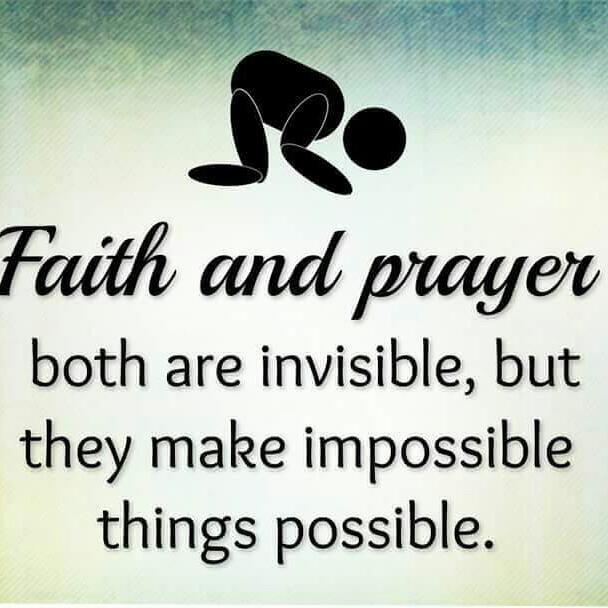The image features a square background with a gradient that transitions from blue at the top to white towards the bottom. The background texture reveals subtle diagonal lines, giving it a grainy or twill fabric-like appearance. At the center of the image is a geometric, black human figure depicted kneeling in prayer. The figure is simplified into shapes, with a separate circular head and oval shapes representing the body, arms, and legs, giving it a digital or abstract feel. Below the figure, bold black text reads "Faith and Prayer," followed by a line of regular black text that states, "Both are invisible, but they make impossible things possible." The arrangement and text suggest that this image is conveying a motivational or inspirational message.